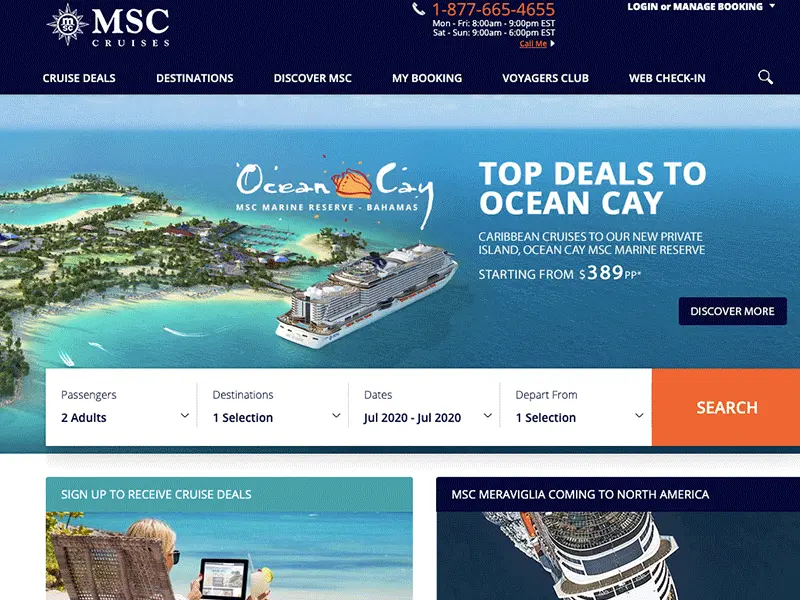This screenshot, captured likely from a laptop, features the homepage of the MSC Cruises website in landscape mode. In the upper left-hand corner, the MSC Cruises logo is prominently displayed. At the upper center, an orange-highlighted phone number, 1-877-665-4655, is accompanied by a phone icon, indicating customer service hours: Monday through Friday from 8 a.m. to 9 p.m. Eastern Standard Time and Saturday to Sunday from 9 a.m. to 6 p.m. There is also a "Call Me" button, which is a clickable link allowing users to request a callback.

In the upper right-hand corner is an option to "Login or Manage Booking." Directly below this section, set against a blue background, are navigation links in white text: Cruise Deals, Destinations, Discover MSC, My Booking, Voyagers Club, Web Check-in, and a search bar.

Dominating the main part of the page is a large, stunning image of an ocean scene. This image features a blue sky overhead and, on the left side, a multi-layered island with a visible coastline where an MSC cruise ship is docked. Overlaid text on the image reads: "Ocean Cay MSC Marine Reserve Bahamas" and "Top Deals to Ocean Cay." The overall layout of the page is designed to guide users in discovering cruise deals and planning their next voyage.